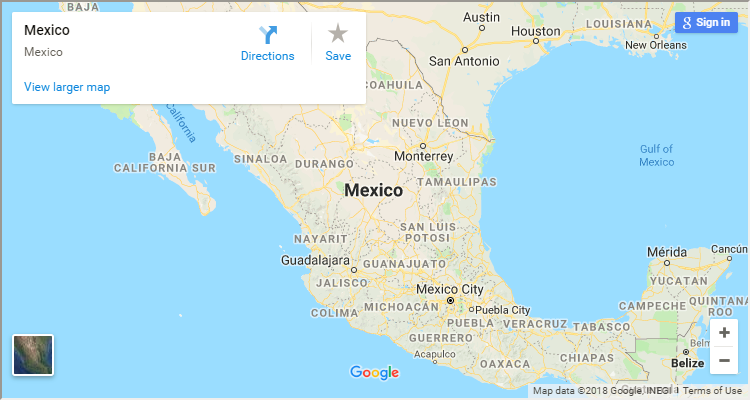In this image, we are viewing a detailed segment of the Google Maps interface focused on Mexico. Prominently featured is a map highlighting various regions and cities within Mexico, all meticulously displayed. In the top left corner, a white information block labeled "Mexico" in bold black letters is present. This block includes clickable options such as "View Larger Map" in blue text, a directions button, and a star icon for saving locations.

In the top right corner of the image, the "Google Sign In" prompt is visible, providing user access to personalized map features. The central portion of the map prominently displays the country's name, "Mexico," also in bold black letters, surrounded by major cities including Guadalajara, Mexico City, Oaxaca, Chiapas, Tabasco, and Yucatán.

The map illustrates significant geographical features, delineating the Pacific Ocean on the western side and the Gulf of Mexico to the east. Various roadways can be seen interconnecting these cities, showcasing the extensive network within and beyond Mexico's borders. Additionally, the map extends northwards, offering a glimpse into the southern United States, including parts of Texas—with cities like San Antonio, Austin, and Houston—and further east to New Orleans in Louisiana. These locations are also interconnected by visible roadways, highlighting the connectivity and geographic scope covered in this illustrative map.